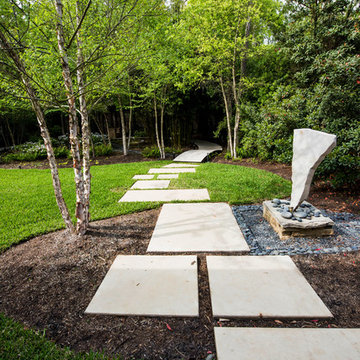The image depicts a meticulously designed outdoor space that could be part of an affluent residence or a small park. The central focus is a walkway made of large, flat, white or cream-colored stone slabs, which are staggered and run from the bottom of the image up to the top, eventually disappearing into a darkened forested area. This path traverses various terrains, including a brown mulchy garden bed, patches of manicured grass, and an archway-like entrance into the woods. 

On the right-hand side of the image, there is a striking stone sculpture resembling an upside-down triangle with rough, slightly bent edges, resting on a rock platform surrounded by smooth, gray circular stones. In the distance, a small raised bridge is visible. The landscape is dotted with trees, including some birch trees in the foreground and more densely-leaved, darker trees further back, contributing to the shaded, mysterious ambiance as the path leads into the wooded area.